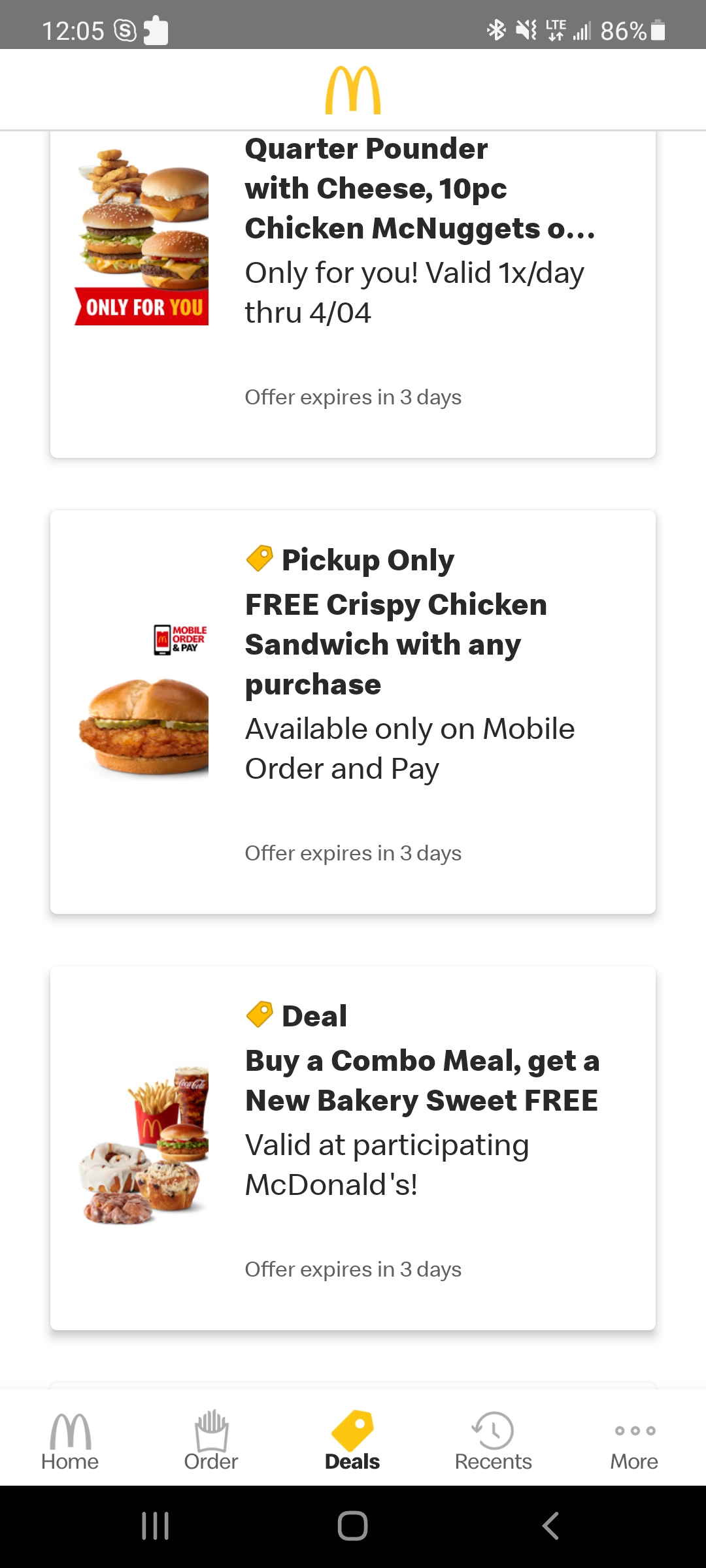This screenshot from a mobile phone captures the display at 12:05, featuring a detailed status bar at the top. From left to right, the status bar presents the time "12:05," followed by a series of icons: a circular 'S' icon, a puzzle piece, a Bluetooth symbol, a speaker with a line through it indicating mute, the "LTE" indicator, a mobile signal strength icon, "86%" for the battery level, and a battery icon. Below the status bar is the main screen, which appears to be the McDonald's app interface.

Prominently displayed at the top of the app screen is the McDonald's logo, characterized by a golden "M." Beneath the logo is a horizontal gray line, followed by a series of vertically arranged white boxes containing promotional coupons.

The first coupon prominently features "Quarter Pounder with Cheese" in black font, along with an enticing image of three Quarter Pounders. The text indicates the offer is exclusive, "Only for you," and remains valid for one day through 4/04, expiring in three days.

The second coupon, labeled "Pick Up Only," advertises a free crispy chicken sandwich with any purchase. This offer is specifically available through mobile order and pay and also expires in three days. Accompanying the text is a mouth-watering image of the crispy chicken sandwich itself.

Overall, the screenshot captures a well-organized McDonald's app featuring time-sensitive deals and clear, detailed promotional information.